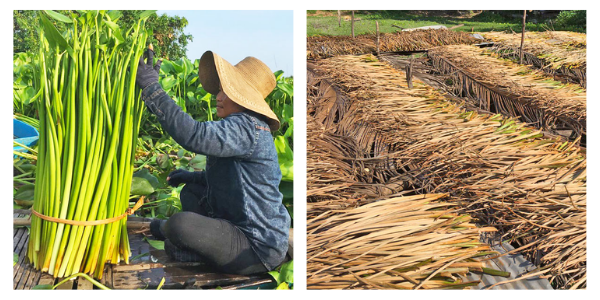The image is a rectangular photograph, wider than it is tall, divided into two square sections by a white line. The left section depicts a woman sitting in front of a bundle of tall green stalks, possibly bamboo or sugarcane, tied together with a cream-colored band made from dried plant material. The woman, clothed in a blue denim shirt, gray pants, and a straw sun hat, appears to be working with the stalks. The greenery and a dark area where she is seated form the background, emphasizing the height of the stalks which tower above the woman even with her hat on.

The right section contrasts by showcasing dried-out stalks of the same plant, now a light brown color. These stalks are laid flat in parallel rows, and while most are brown, some retain a hint of green, indicating they have been drying out in the sun for quite some time. The background contains patches of green grass, indicating a farming area where the plants are being processed and dried.